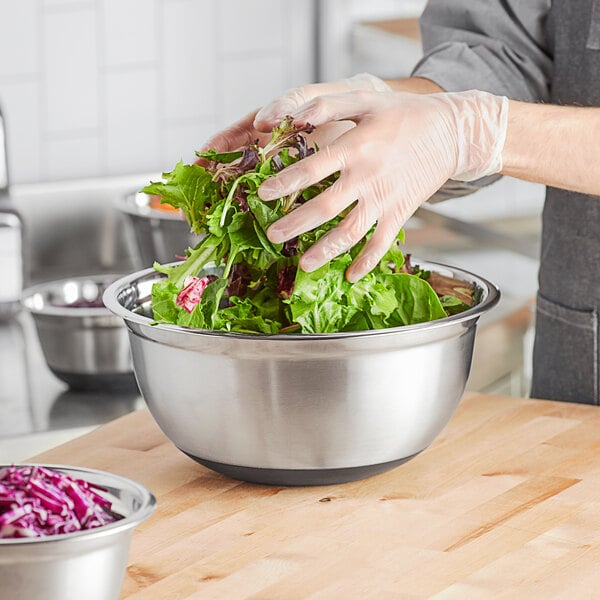In an industrial kitchen, a photograph captures a chef—identified by their gray long-sleeve shirt and dark gray apron—vigorously tossing salad greens in a large silver bowl using translucent latex gloves. The bowl rests on a light wooden butcher block counter, next to another smaller bowl filled with finely chopped red cabbage. The chef's hands lift the salad, which includes romaine, iceberg, and red-tinted crunchy greens, showcasing the meticulous mixing process. In the blurred background, white walls and stainless steel countertops are adorned with additional empty silver bowls and hints of orange ingredients. The scene evokes a sense of professional culinary preparation amidst a clean, organized kitchen environment.